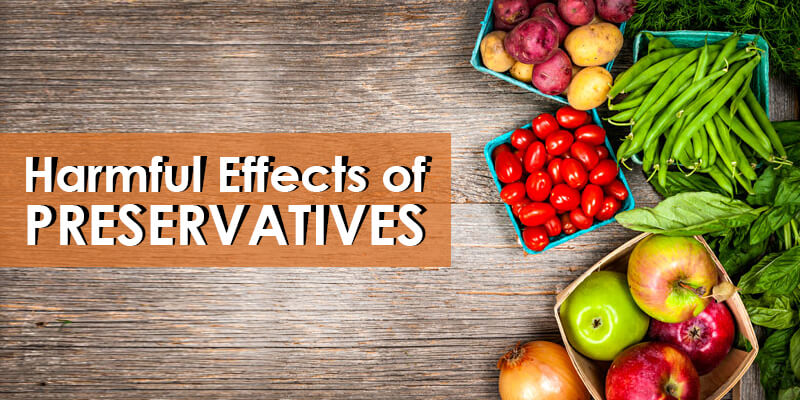The image appears to be a magazine or pamphlet page featuring the title "Harmful Effects of Preservatives" in white text on a brown bar, which is centered vertically on the left side of the image. The background is a well-weathered wooden table with a grayish-tan, grainy texture. On the right side of the page, there are several blue square containers filled with a variety of fruits and vegetables. Starting from the top left and moving clockwise, there is a container of mixed yellow and red potatoes, followed by a container of string beans. Below the green beans, a container holds a mix of red and green apples. Next to the apples, but not in a container, lies a single large yellow onion. Below the string beans container is a another container with cherry tomatoes. An additional note of green basil leaves is positioned near the bottom right edge of the image, outside of any container. The organized layout and the rustic setting create a strong visual contrast between natural produce and the warning about preservatives.